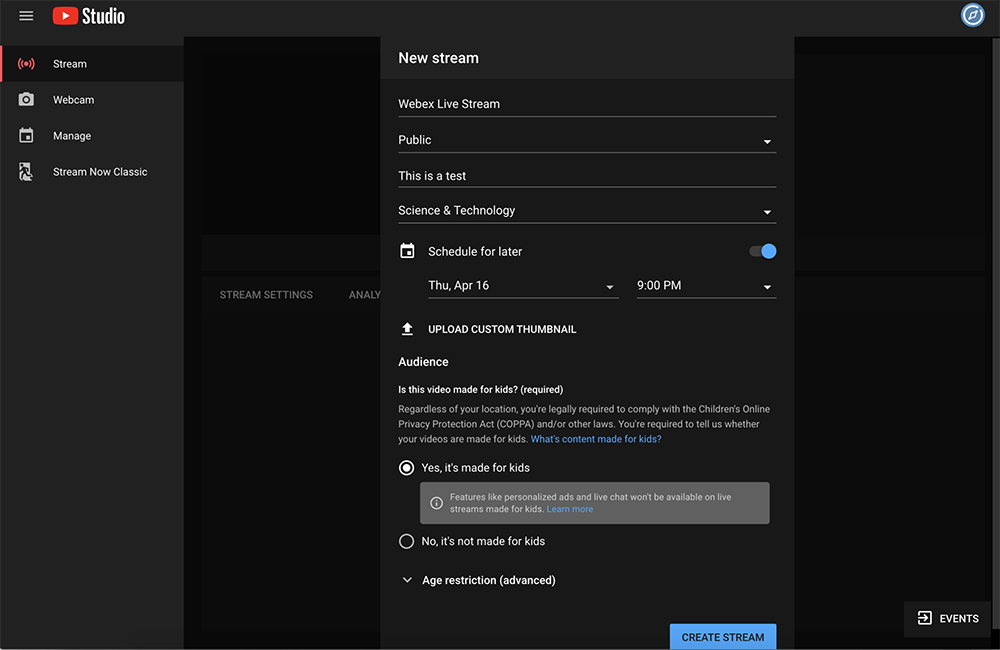The image appears to be a screenshot of a YouTube Studio dashboard, likely captured from a computer screen due to its resolution and layout. On the left side of the interface, there is a prominent red square with a white play arrow, indicative of YouTube's branding. Next to this icon, the word "Studio" is visible.

Below this section, the navigation options include "Stream," "Webcam," "Manage," and "Stream now classic." 

In the central portion of the screen, a list is visible displaying a form for creating a new live stream. The form includes fields such as:
- "New stream" 
- "WebEx live stream" 
- "Public"
- "This is a test"
- "Science and Technology"
- "Scheduled for later: Thursday, April 16th at 9 p.m."

There is also an option to "Upload custom thumbnail," which currently displays an image resembling a download icon. 

Further down, there is an audience setting section with the question, "Is this video made for kids?" followed by a parenthetical note indicating this is required. Below this, text explains that regardless of the user's location, they must comply with the Children's Online Privacy Protection Act (COPPA) and other similar laws, and are required to specify whether their video is made for kids. 

A clickable link titled "What's content made for kids?" is seen in blue, providing additional information for the user. 

Finally, a section indicating the video has been marked as "Yes, it's made for kids" is completed. The "Create stream" button is shown in blue at the bottom of the interface.